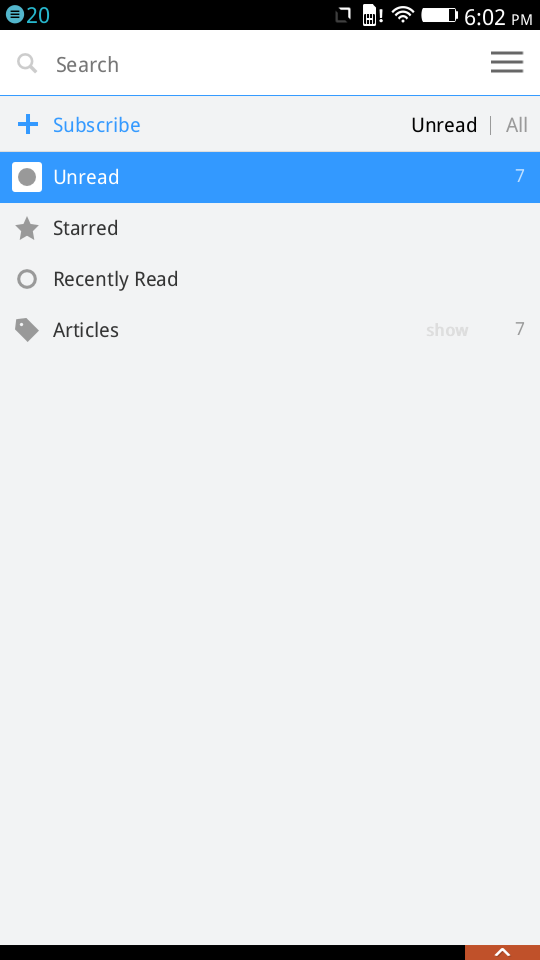This screenshot from a phone displays a multi-colored interface with several icons and notifications. The top quarter-inch of the screen is black, followed by a white segment, and then the remaining part is a light bluish-gray. In the top-left corner, a small blue circle features three black lines and the number 20 in blue. On the right side, the time is displayed as 6:02 p.m. in white. 

The status bar shows a battery icon that is three-quarters full, a fully connected Wi-Fi symbol, a rectangle with an exclamation point, and a multi-colored square icon. The square is white on the top-right and gray on the bottom-left, and within the white part, there is a search icon and the word "search" in black. To the right, three black lines are visible. 

A thin, light blue border separates this area from the main interface. Below, a blue plus sign is accompanied by the word "subscribe" and to the right of it, "unread" is written in black with a gray slash. Further down, a white square with a central gray circle reads "unread" in white, and the number seven appears on the right. 

A dark blue rectangle spans the screen, below which various interface elements are listed: a gray star followed by "starred" in black, a gray circle with "recently read" in black, a gray sales tag icon with "articles" in black, and another number seven on the right.

At the very bottom, a thin black border extends until the right corner, which is marked by an inch of orange with a white greater-than sign pointing upward.